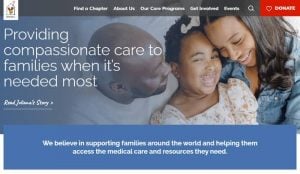**Website Banner Image Description:**

At the top of the image, there is a banner from a website, albeit shown on a small scale. In the upper left-hand corner, a logo enclosed in a white box is visible, though its details are unclear—it seems to be in the shape of a house. Next to the logo, there are navigation links that read: "Find a Chapter," "About Us," "Our Care Programs," "Get Involved," and possibly "Events." A white magnifying glass icon signifies the search function. Adjacent to that is a red block containing a white heart and a white "Donate" button.

Beneath these navigation links, a tagline reads, "Providing compassionate care to families when it needed most," accompanied by a call-to-action link, "Read Julian's Story."

The main image features three individuals: a young man in a white shirt, a young woman with brown hair wearing a denim jacket, and a young girl with a bow in her hair and a tan-colored dress.

At the bottom of the banner, a blue strip with white font declares, "We believe in supporting families around the world and helping them access the medical care and resources they need."